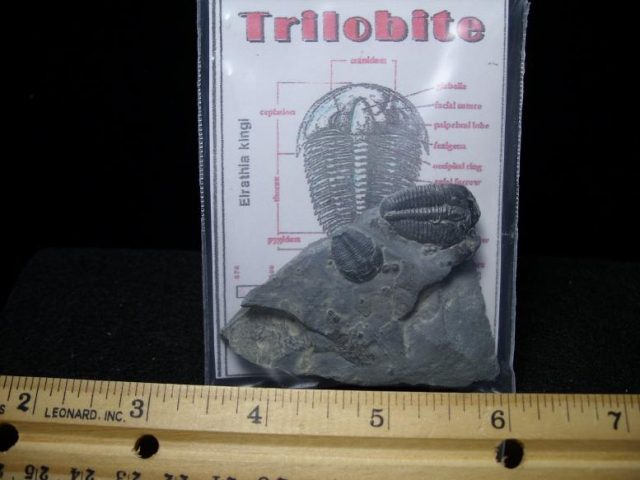In the image, a fossilized trilobite is prominently displayed on a rock, laying on top of a wooden ruler that measures from 2 to 7 inches, indicating the rock's width is approximately 5 inches. The trilobite fossil exhibits ridged, spiky features and is placed in front of a detailed informational card. This card, set against a solid black background, reads "trilobite" in red letters at the top. Below, it features a black-and-white illustration of the trilobite with various parts labeled in red. The card also includes the scientific name "Elrathia kingii." The fossil and educational card together create a detailed and informative presentation of the trilobite, capturing both its physical characteristics and scientific classification.